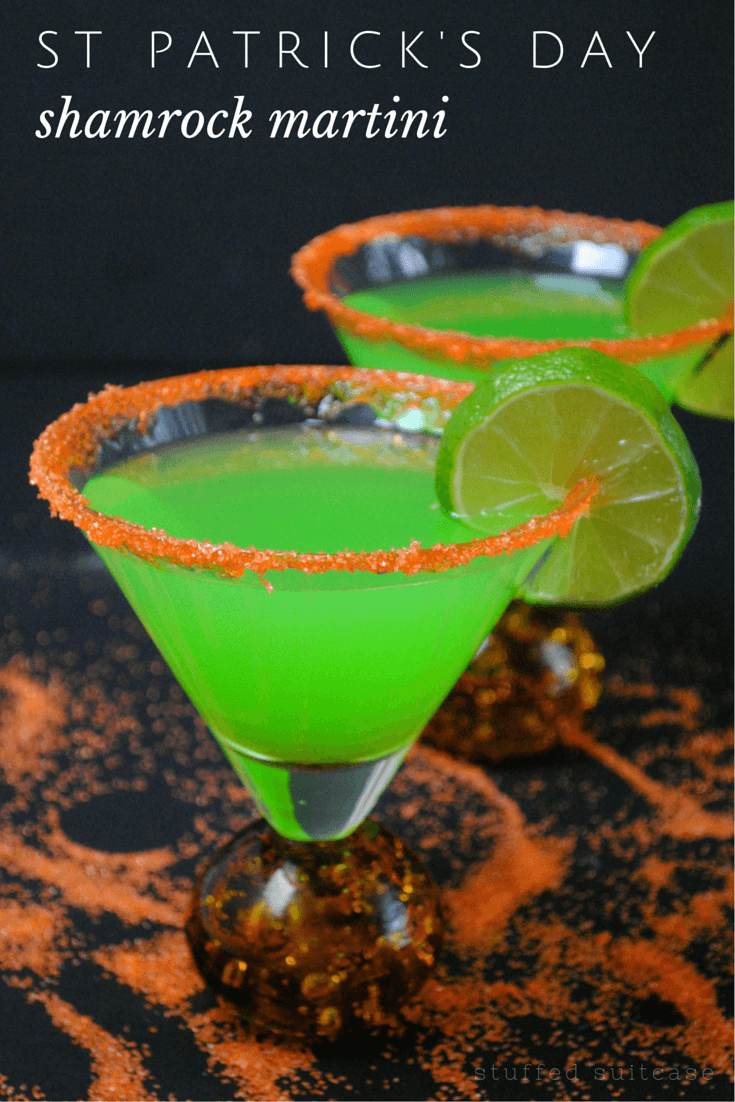This image, likely intended for a recipe or bartending site, showcases a vibrant St. Patrick's Day advertising poster featuring Shamrock Martinis. The background is a black marble-like counter accented with orange patterns. In white lettering at the top, the text "St. Patrick's Day" and "Shamrock Martini" prominently announce the festive theme. 

The scene displays two martini glasses, one positioned prominently in the foreground and the other slightly in the background. Each glass contains a bright, lime green liquid, adding a fluorescent pop of color to the composition. The rims of the glasses are adorned with granulated orange sugar, creating an eye-catching contrast. Both martinis are garnished with a lime slice perched on the rim, further enhancing the visual appeal.

The overall arrangement captures a rich palette of greens, oranges, blacks, and whites, bringing a festive and colorful charm to the viewer, perfectly embodying the spirit of St. Patrick's Day.